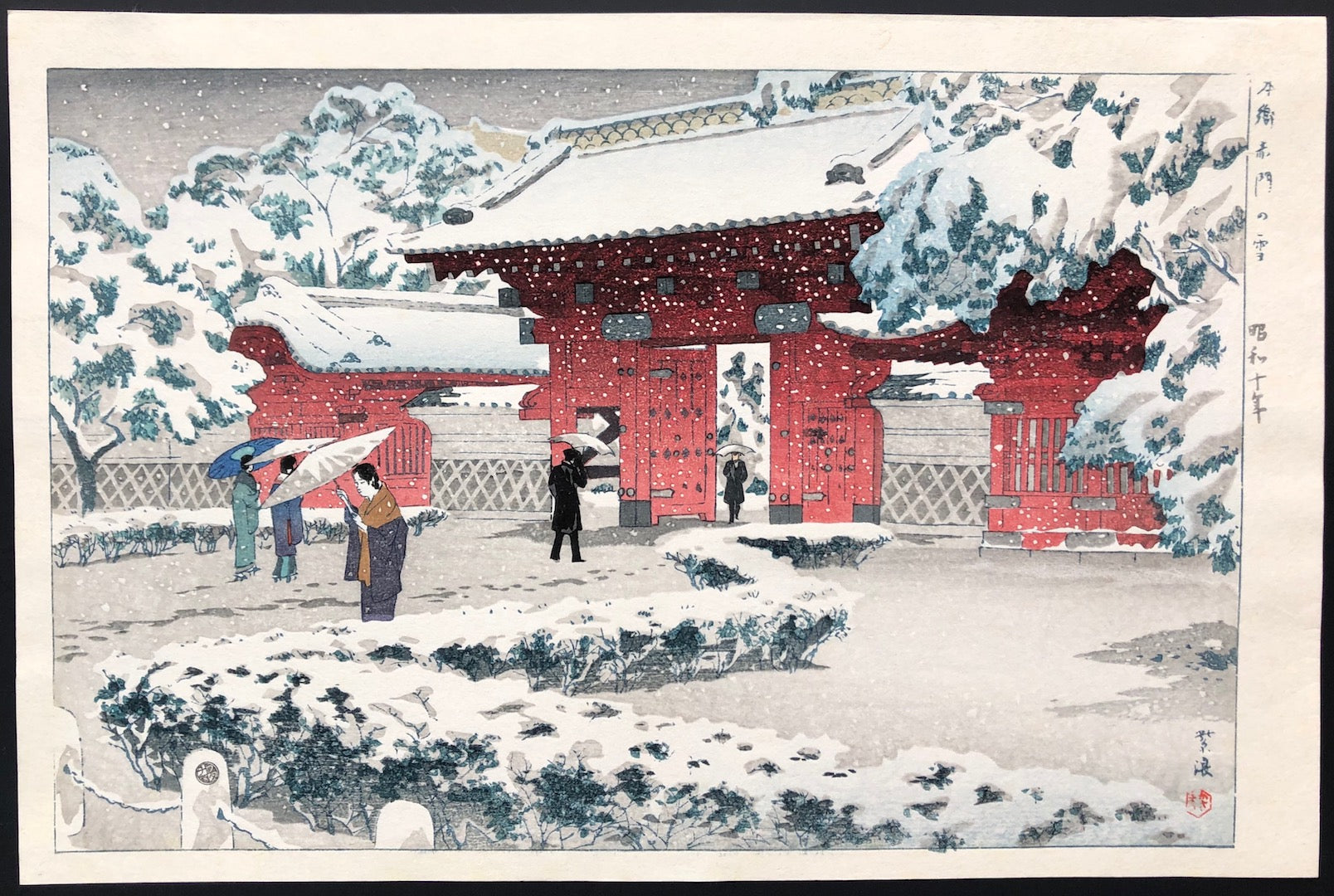This color illustration, framed in a plain black frame with a cream-colored mat, depicts a picturesque wintry scene centered on a traditional Asian architectural structure. The building, adorned with Asian characters vertically on the right side of the mat and near the bottom right corner of the artwork, showcases a classic pagoda-styled roof covered in snow. Its slightly curved roof and red color evoke the serene beauty of traditional Asian temples or gates. 

The scene unfolds along a snow-covered pathway lined with shrubs and zigzagging hedges blanketed in thick snow. To the sides of the pagoda, large trees stand heavy with snow. A distinctive feature is the post and chain fencing along the lower left of the image. The pathway is animated by five people holding various umbrellas to shield themselves from the falling snow. Most umbrellas are white, but one stands out in blue with a small green patch. The figures include both men, dressed in black coats and pants, and women, attired in vibrant kimonos, with one woman notably wearing a long purple kimono and a gold wrap.

This exquisitely detailed artwork captures a serene outdoor setting during winter, providing a harmonious blend of nature and traditional architecture under a snowy landscape.